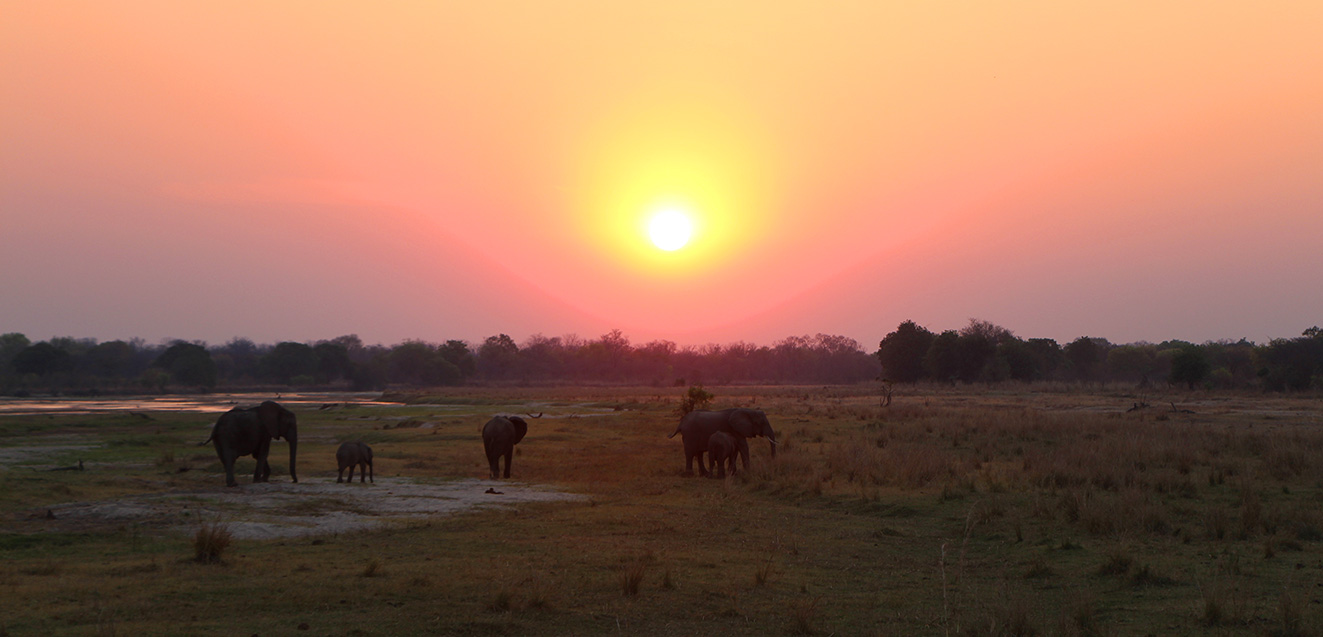In this beautiful, picturesque scene likely taken in a natural wilderness setting such as South Africa, the sky paints a mesmerizing gradient: vibrant yellow surrounding a radiant sun at the top, shifting to pinkish hues in the middle, and finally transitioning to a deeper, grayish purple near the horizon. The sun, beaming warmly, casts a gentle halo and illuminates the landscape beneath. Below the colorful sky, a range of pink and gray clouds adds depth to the horizon, which is fringed with a line of diverse trees.

Dominating the forefront is a lush, green field adorned with various plants. In the midst of this verdant terrain, a family of five elephants roams freely. The scene captures both an adult and a baby elephant prominently in the center, while another adult stands further back with its rear facing the viewer. Towards the right, an additional adult elephant stands beside a nursing calf. Each elephant varies significantly in size, highlighting the presence of both young and mature individuals. The overall tranquility of the photo is enhanced by what appears to be a small pond and the vast spread of nature, truly encapsulating the serenity and raw beauty of the wild.